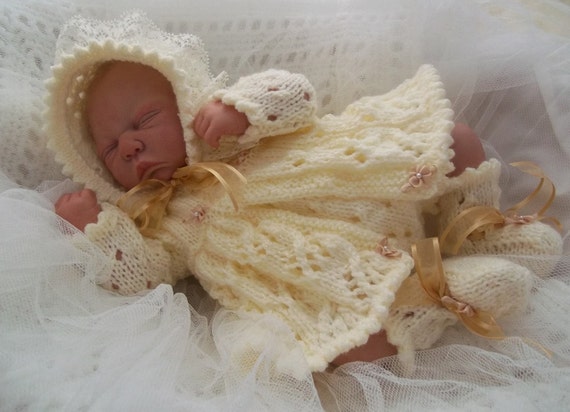This image captures a heartwarming close-up of an infant baby girl sound asleep, lying on her side with her face to the left and her feet to the right. She is clad in a handmade, intricately hand-knit ivory outfit, consisting of a long-sleeved jacket adorned with a lace-embellished hood, and matching booties. The ensemble is also detailed with delicate pink flowers and tied together with a beautiful ribbon under her chin, which echoes the ribbons on her mid-calf booties. Her little fists are raised beside her face, accentuating her slightly frowning, yet peaceful expression. The baby is resting on a soft, crocheted white blanket covered with layers of white tulle and surrounded by silken textures, including gold silk bows around her booties, adding to the overall elegant and serene composition of the photograph.